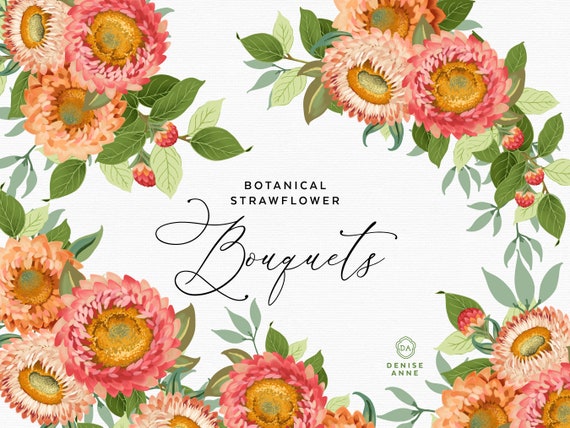The image is a vividly designed book cover titled "Botanical Strawflower Bouquets." Displayed in small, black block letters, the title stands prominently at the center on a clean white background. Below this title, in a larger cursive font, the word "Bouquets" gracefully enhances the aesthetic. Stylishly framing the four corners of the cover are clusters of strawflowers in varying shades of peach, red, pink, and a very light salmon color, each accented with dark green and light mint green leaves that feature visible veins. The floral pattern includes additional botanical elements such as berries, possibly raspberries or strawberries, contributing to the lush and vibrant composition. At the bottom right corner, the author's name, "Denise Anne," appears in light green block letters next to a green trefoil-shaped logo with the initials "DA." Overall, the imagery and detailed botanical accents create a captivating and elegant presentation.